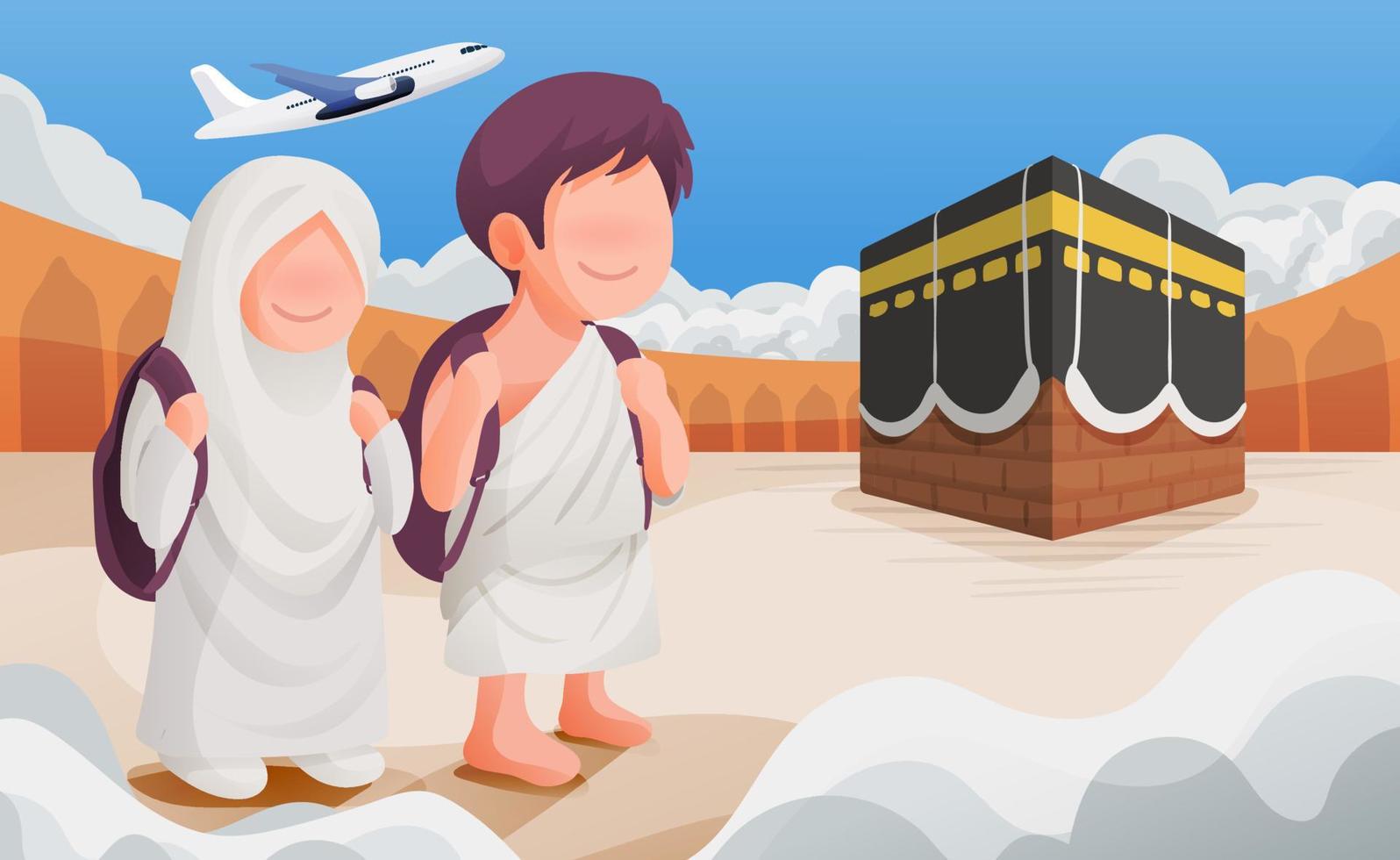In a simple digital cartoon drawing, two young figures—a male and a female—stand in a large courtyard that resembles an open coliseum-like space. On the right side, there is a distinctive black structure that appears to be the Kaaba, surrounded by a few doors and brick accents. The male, with brown hair and bare feet, is dressed in a white toga and carries a purple backpack. The female, wearing a white burqa and white shoes, also has a purple backpack. Both figures have unusually smooth faces with only smiling mouths and no other facial features. Above them, an airplane is taking off, angled upward into a blue sky.